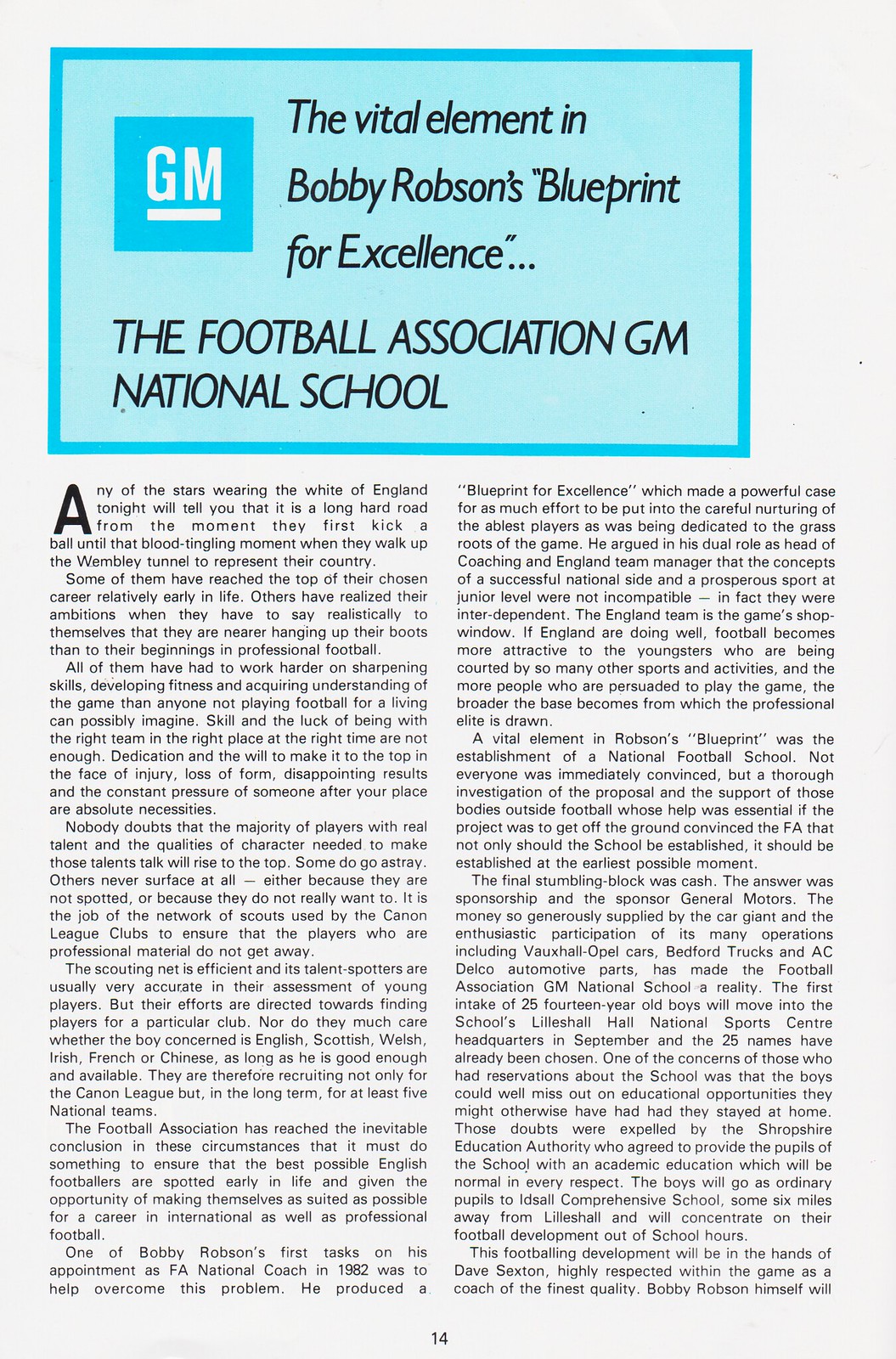The image depicts page 14 of a book or newspaper, featuring an article titled "The Vital Element in Bobby Robson's Blueprint for Excellence" with a focus on "The Football Association GM National School." At the top, there is a light blue rectangle with a dark blue border, containing a darker blue square with the white letters "GM" underlined within it. To the right of this square, in black text, is a quote emphasizing the importance of a blueprint for excellence. Below the blue rectangle is the heading: "The Football Association GM National School," written in capital letters and black font.

The body of the article comprises 11 paragraphs explaining the rigorous journey of English football stars from their early days to representing their country, the role of scouts in nurturing talent, and the efforts of Bobby Robson in establishing a national football school. The detailed text discusses the challenges and dedication required to excel in professional football. It also covers the significant sponsorship by General Motors, ensuring the financial success of the Football Association GM National School, the academic provisions for the students, and the key personnel involved in the school's football training. The text ends mid-sentence, indicating more content on the following page. The background of the image is gray, and the page number "14" is centered at the bottom.